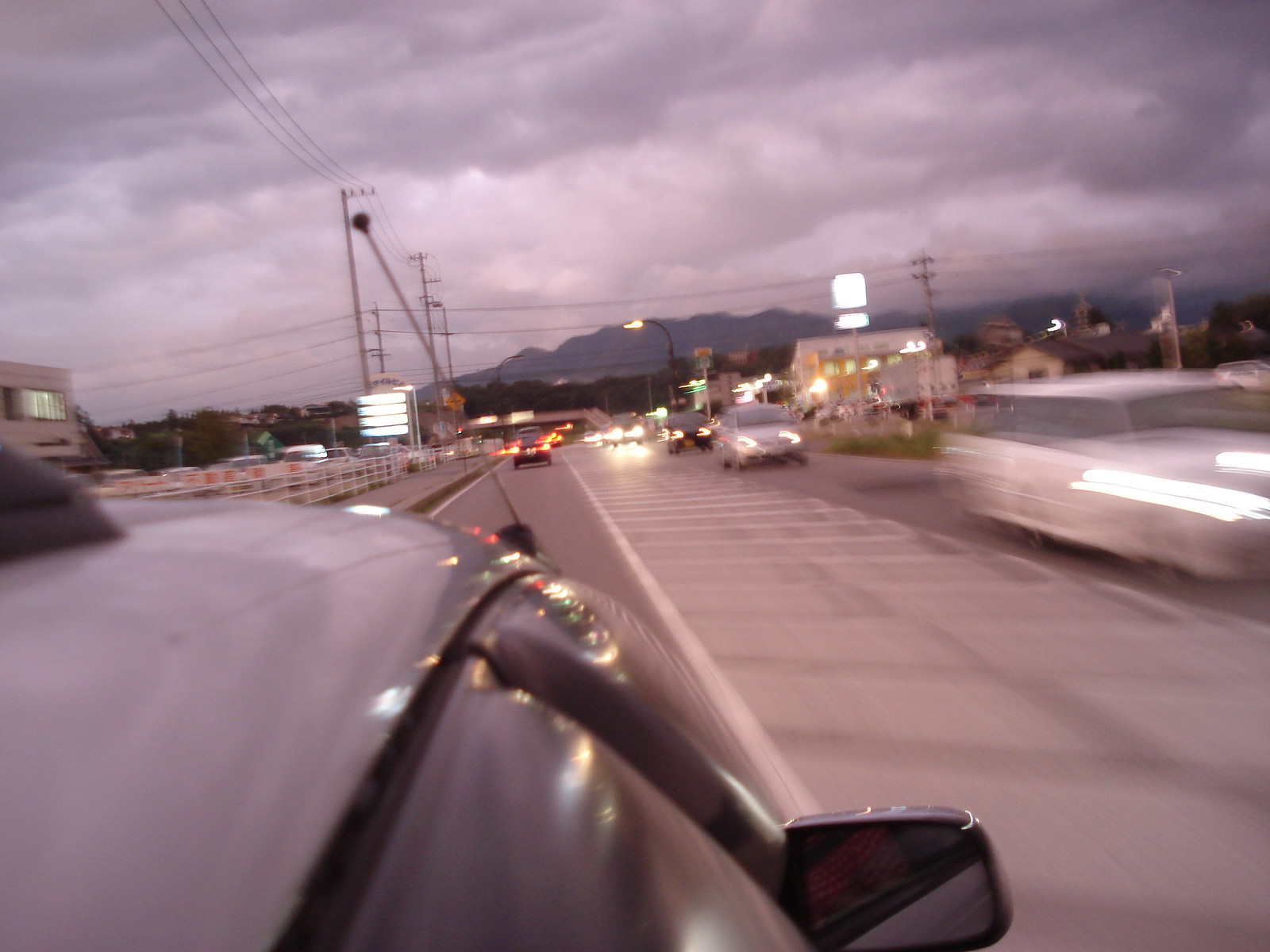The photograph captures a dynamic, stormy scene on what appears to be a two-lane road in England or a similar country where cars drive on the left. The sky is dominated by huge, dark grey clouds that create an ominous atmosphere, lending a monochromatic, grey tone to the entire image as though the white balance has been thrown off by the looming storm. The unique camera angle, seemingly mounted to the roofline of a black car, provides a view of the car's curving roof, passenger window, and side mirror on the right. The scene ahead shows the taillights of a vehicle several car lengths away, with the blurred white hashed road markings indicating that the car is traveling at speed. To the right, the image captures ghosted and elongated headlights of oncoming traffic, while a vehicle just exiting the frame indicates movement in the opposite lane. To the left, there's a railing suggesting the road is on an overpass, and in the distance, power lines and faint outlines of mountains and retail shops can be seen, adding depth to this stormy, night-time road adventure.